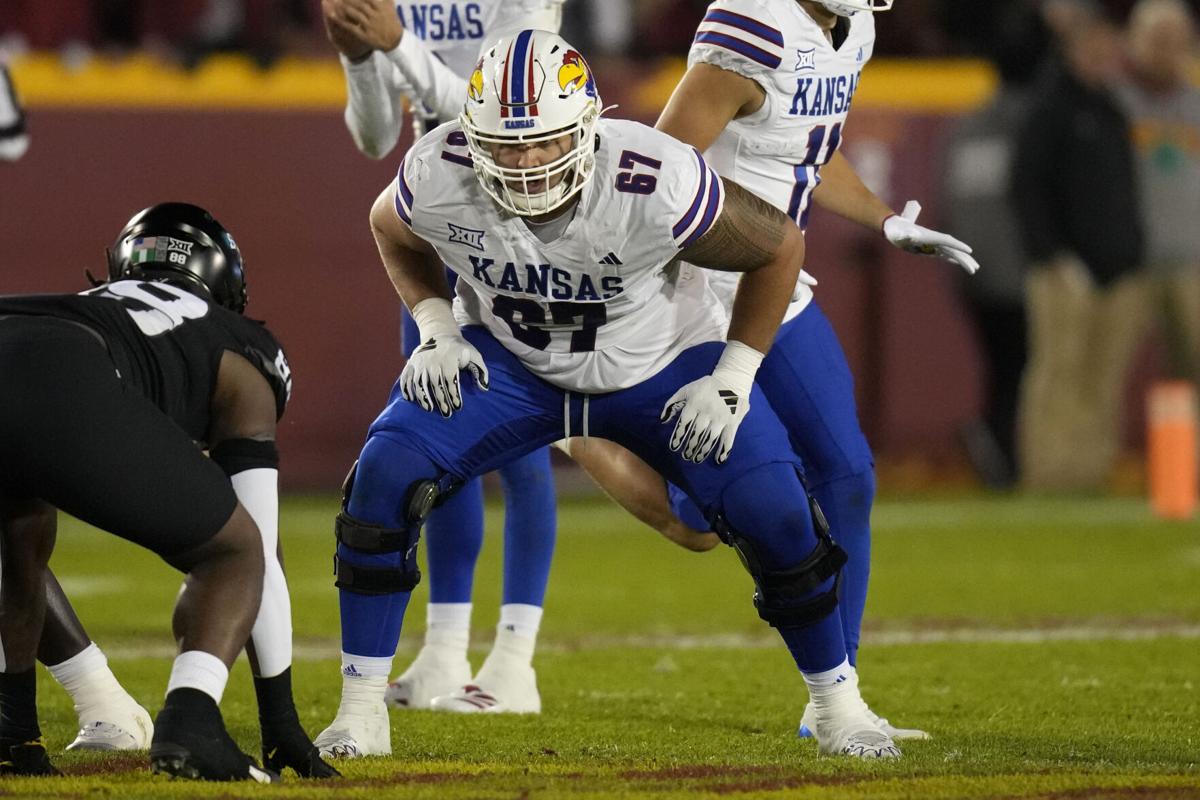The image depicts a tense moment before the snap in an American football game featuring the Kansas Jayhawks. Center stage, player number 67 in a white jersey, blue pants, and white shoes squats in preparation, eyeing his opponent. Directly behind him, number 11, a tall, lanky quarterback, holds the football, ready to initiate the play. Both players' helmets showcase the iconic Jayhawks logo. To the squatting player’s right, another Kansas player is captured in a dynamic gesture, seemingly questioning his teammate.

The opposing team, represented by a player in a fully black uniform adorned with the number 88 on his helmet, remains somewhat indistinct, except for his visible defensive stance. The game unfolds on a verdant green field, marked by an orange pylon near the end zone. The background is slightly blurred, revealing an audience and coaching staff intently watching the action, further emphasizing the game's live and competitive atmosphere.